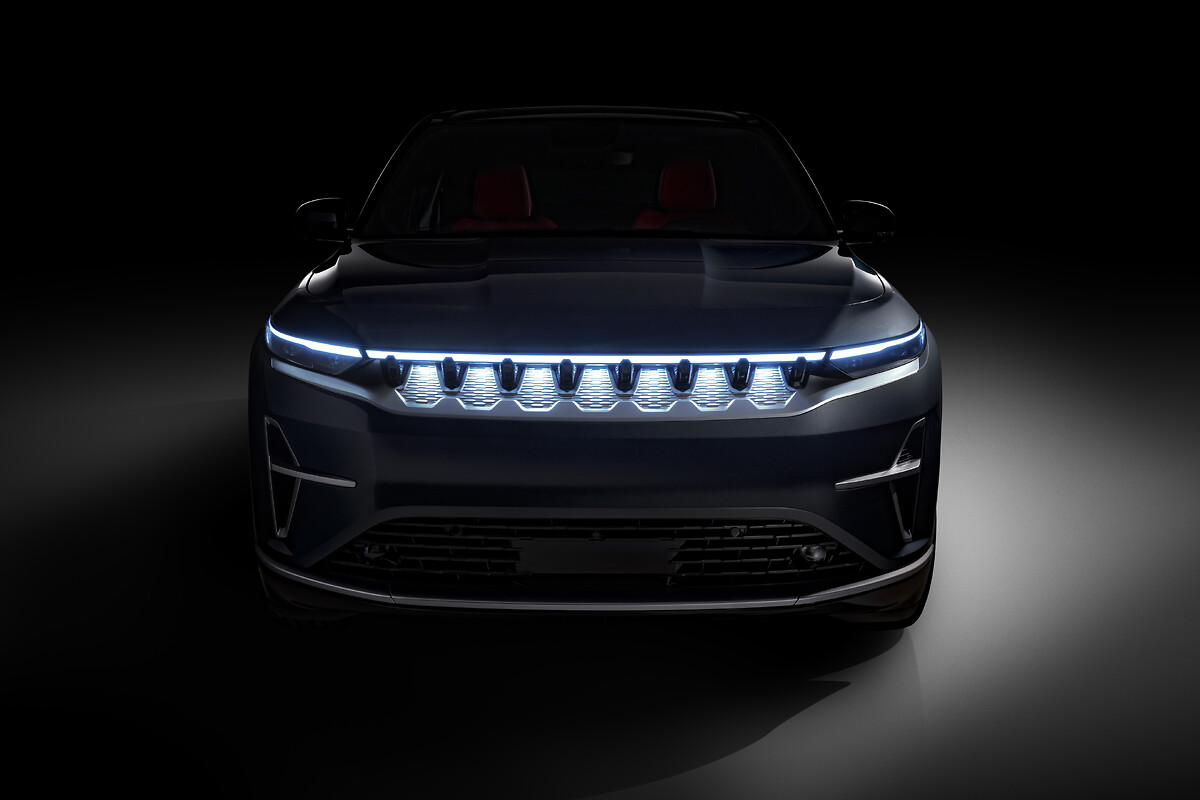A high-end concept car is prominently displayed in the center of a dark, indoor setting, illuminated by artificial lighting that casts a grayish light on the floor. The car, which appears to be a sleek, silverish-blue color, showcases a futuristic design with a seamless front grille and innovative lighting features. Notably, along the edge of the hood, there are nine distinctive blue lights that replace traditional headlights and thin, sleek strip lights that add to the car's modern aesthetic. The windshield offers a glimpse of red seats inside, adding a touch of contrast. The overall backdrop is shrouded in black, enhancing the car’s dramatic and sophisticated appearance.